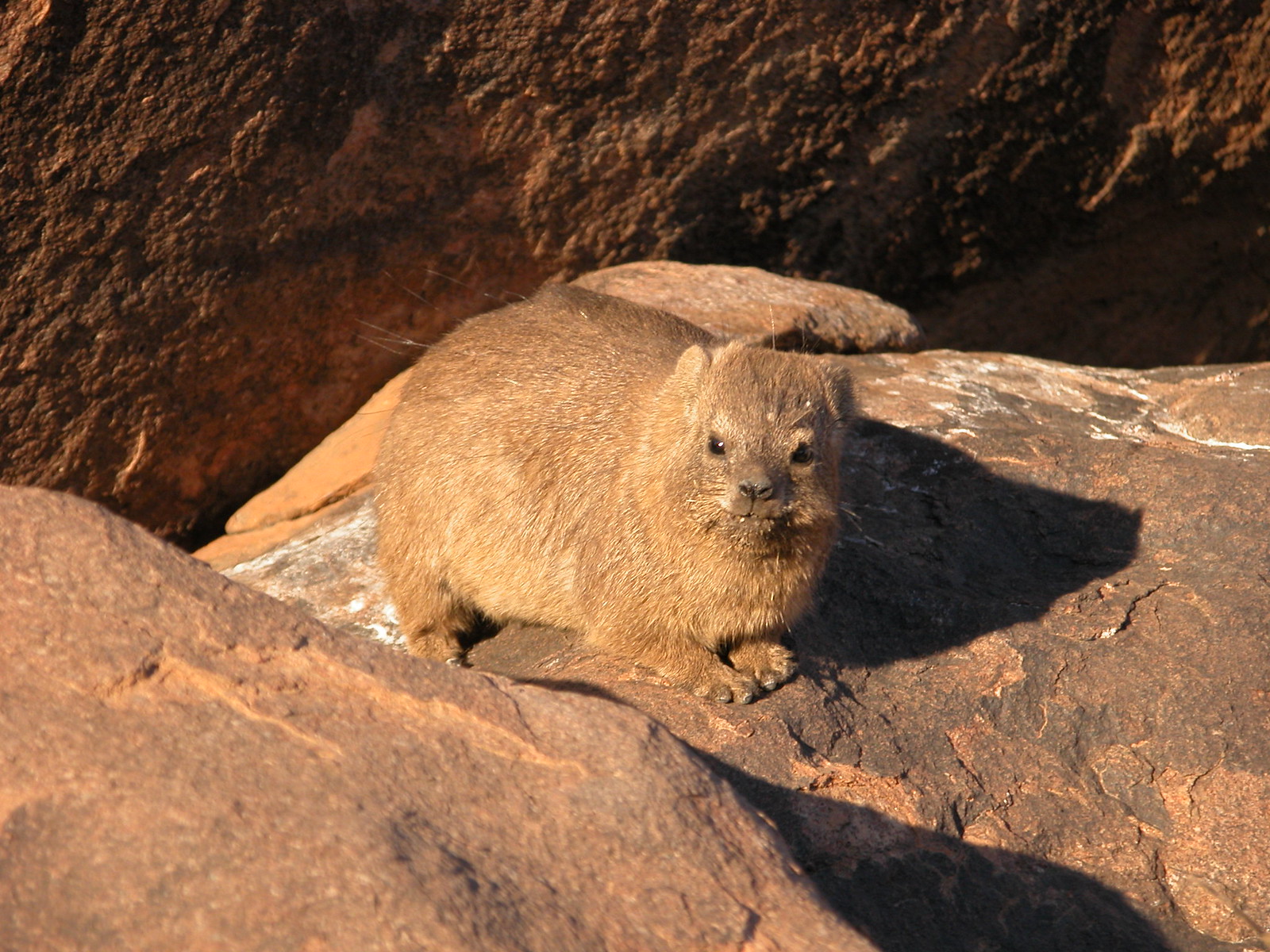This photograph captures a brown animal, possibly a groundhog or an otter, perched on a large, sunlit rock. Its fur, ears, nose, and feet are uniformly brown, blending seamlessly with the similarly hued rock it stands on. The animal’s stance reveals three legs—two in the front and one in the back—with one leg hidden from view. The scene is set against a backdrop of multiple large rocks, including a substantial rock wall that slightly differs in color, being a darker shade of gray and tinged with a hint of rust and white. The setting suggests a natural, possibly desert or rocky beach environment, bathed in bright sunlight.